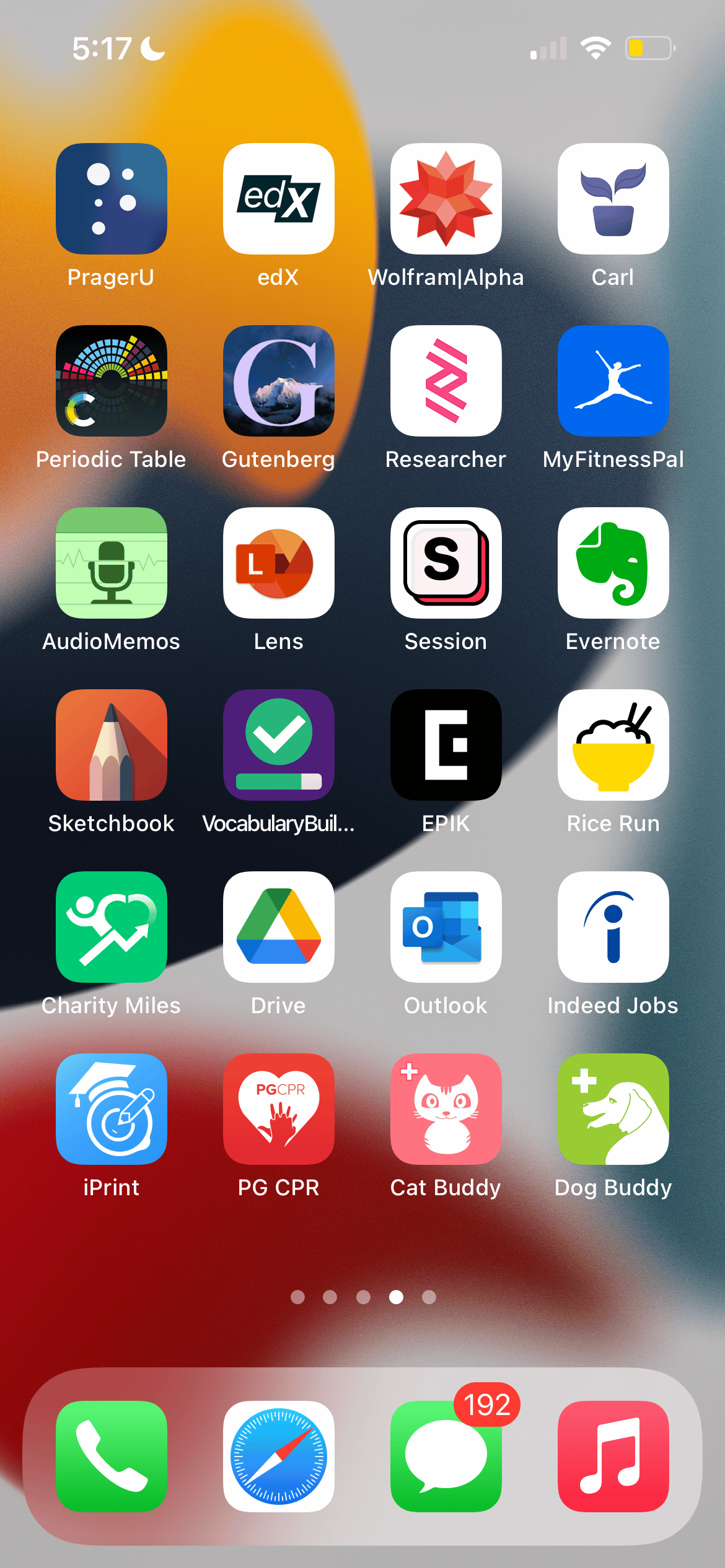This detailed screenshot taken on a smartphone shows the iPhone home screen with various elements visible. The time displayed in the upper left-hand corner is 5:17, accompanied by a moon icon indicating Do Not Disturb mode is activated. The Wi-Fi signal shows only one bar, suggesting a weak connection, and the battery life is critically low, indicated by the orange color.

The home screen features a grid layout containing 24 different apps, organized in sets of four rows across six columns. Beneath these apps, there are five dots, signifying that there are five total pages of apps, with the current view being on the fourth page.

At the bottom of the screen, the standard dock icons are present: the green telephone icon for making calls, the Safari browser icon, the Messages app icon showing 192 unread messages in red, and the Music app icon. The overall layout and visible indicators suggest that the device's user is in need of both charging the battery soon and possibly addressing their numerous unread messages.